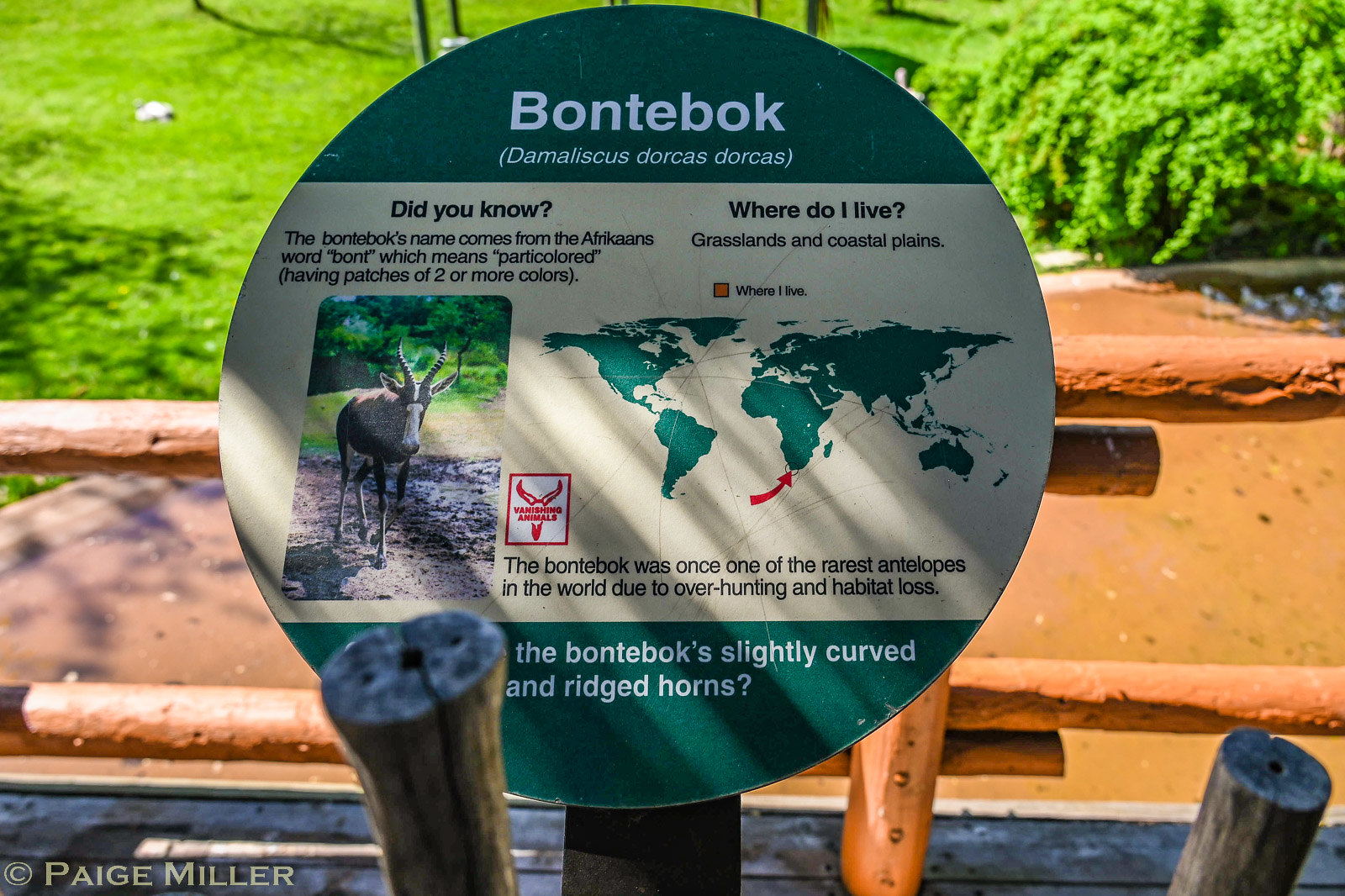This detailed zoo sign describes the Bontebok, an antelope species with the scientific name Demoliscous Dorcus Dorcus. The sign is circular, with green borders at the top and bottom, and an off-white background in the center. The top green section reads "Bontebok" in bold white text, followed by the scientific name in parentheses. Below, it states, "Did you know the Bontebok's name comes from the Afrikaans word 'bont,' which means party-colored, having patches of two or more colors?" 

Accompanying this text, a detailed illustration of the Bontebok is positioned to provide a visual reference. To the right, the sign asks, "Where do I live?" and answers with "Grasslands and coastal plains," alongside a world map pinpointing South Africa in a small orange section. Additional information notes that the Bontebok was once one of the rarest antelopes due to overhunting and habitat loss, and mentions its slightly curved, high-ridged horns. The bottom left corner credits photographer Paige Miller. 

The sign is mounted on a wooden fence, with horizontal beams behind it, suggesting an elevated viewing area at the zoo, possibly above a pond with surrounding grass and bushes.